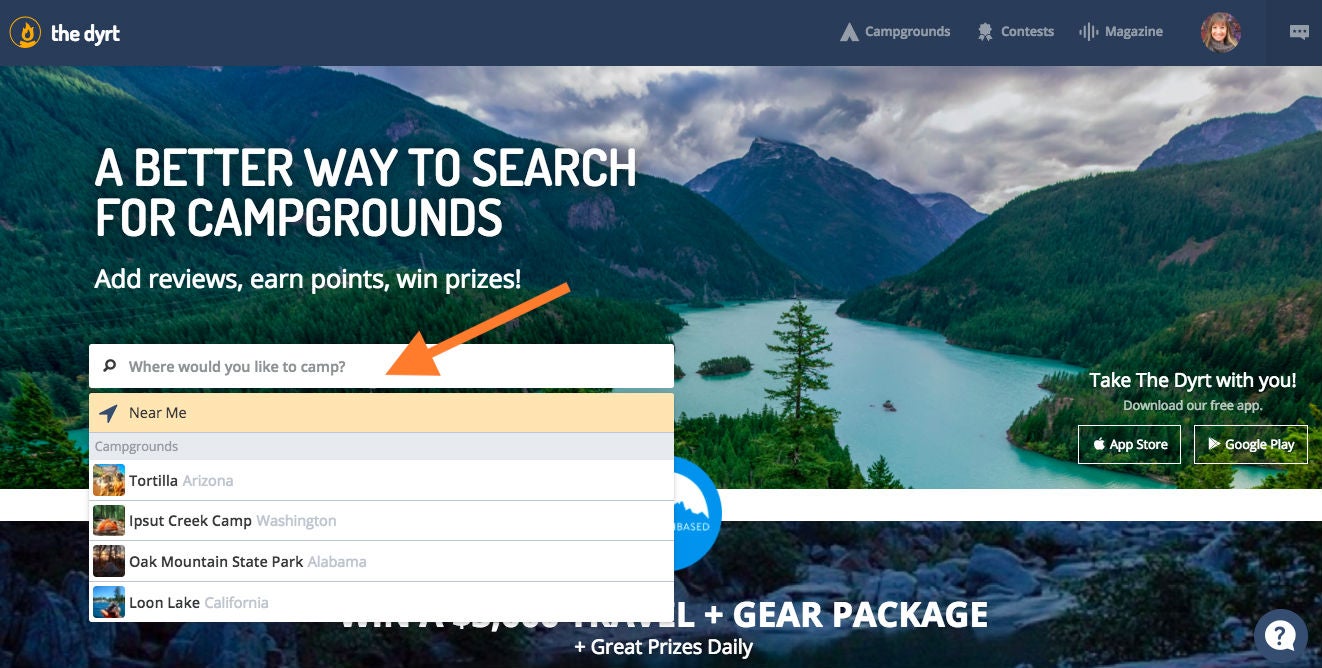Explore The Dyrt: The Ultimate Camping Resource

The screenshot showcases The Dyrt’s homepage, an innovative platform designed for camp enthusiasts to search for campgrounds, add reviews, earn points, and win prizes. At the top of the screen is a search bar, offering quick access to campsite information. Before any input is entered, the page suggests popular campgrounds, including Tortilla in Arizona, Ipsut Creek Camp in Washington, Oak Mountain State Park in Alabama, and Loon Lake in California. The interface utilizes a dark blue color scheme with varying shades of gray font, creating a visually appealing and user-friendly experience. Notably, a user is signed in, as indicated by a woman's profile picture. The homepage features a stunning main image depicting a serene river meandering through lush, green mountains, embodying the essence of outdoor adventure and natural beauty.